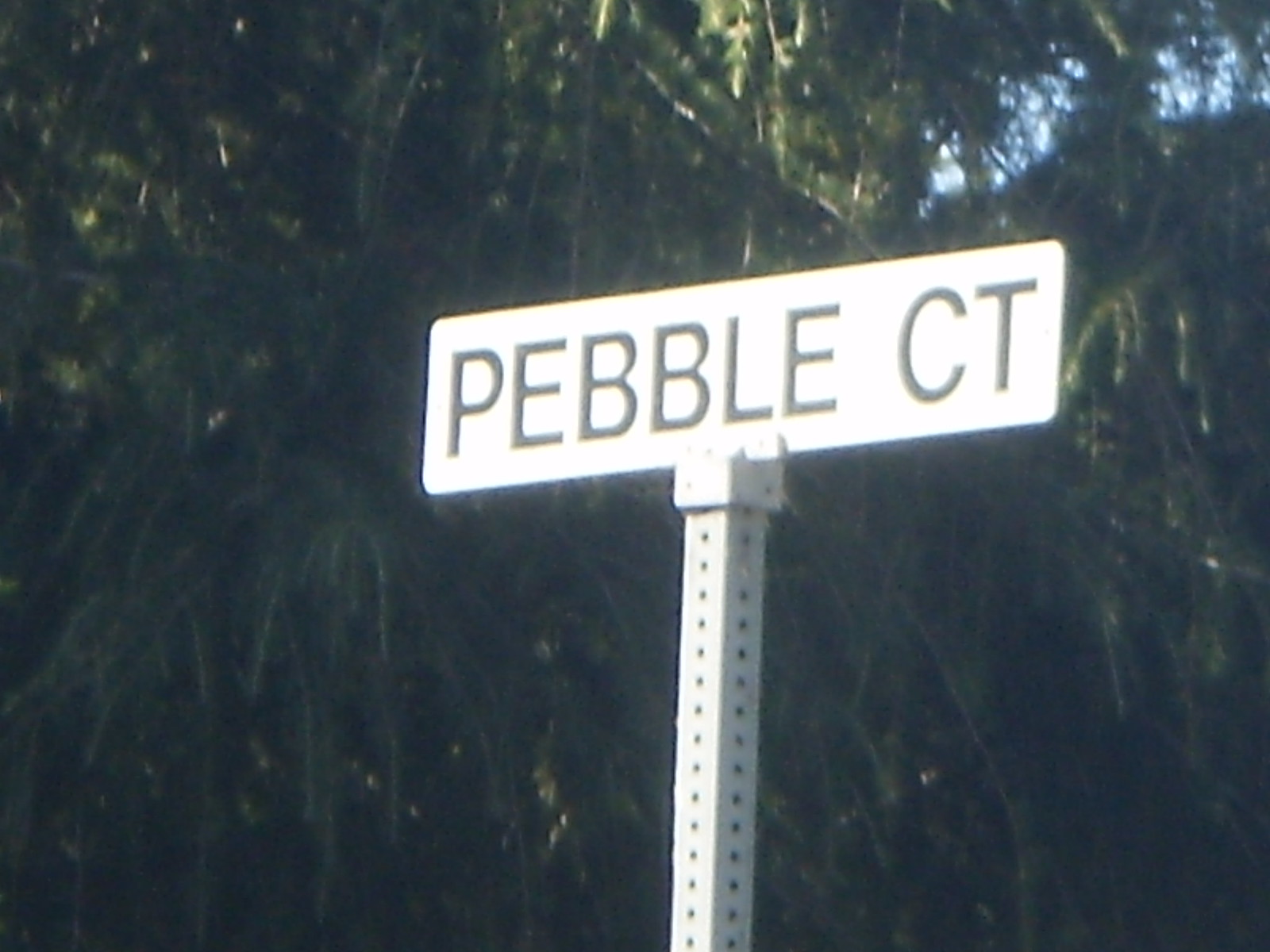In this vibrant outdoor scene captured on a bright, sunny day, a cluster of lush green trees fills the background, their densely packed foliage providing a verdant backdrop. A sliver of clear, blue sky peeks through in the upper right-hand corner, adding a touch of contrast to the greenery. Dominating the center of the image is a street sign, securely mounted on a square, perforated metal pole. The sign, white with bold black capital letters, caps the top of the utilitarian pole, which features evenly spaced holes along its length. The sign prominently displays the name "Pebble Court," with "Court" abbreviated as "CT," clearly indicating the street name to any passerby.